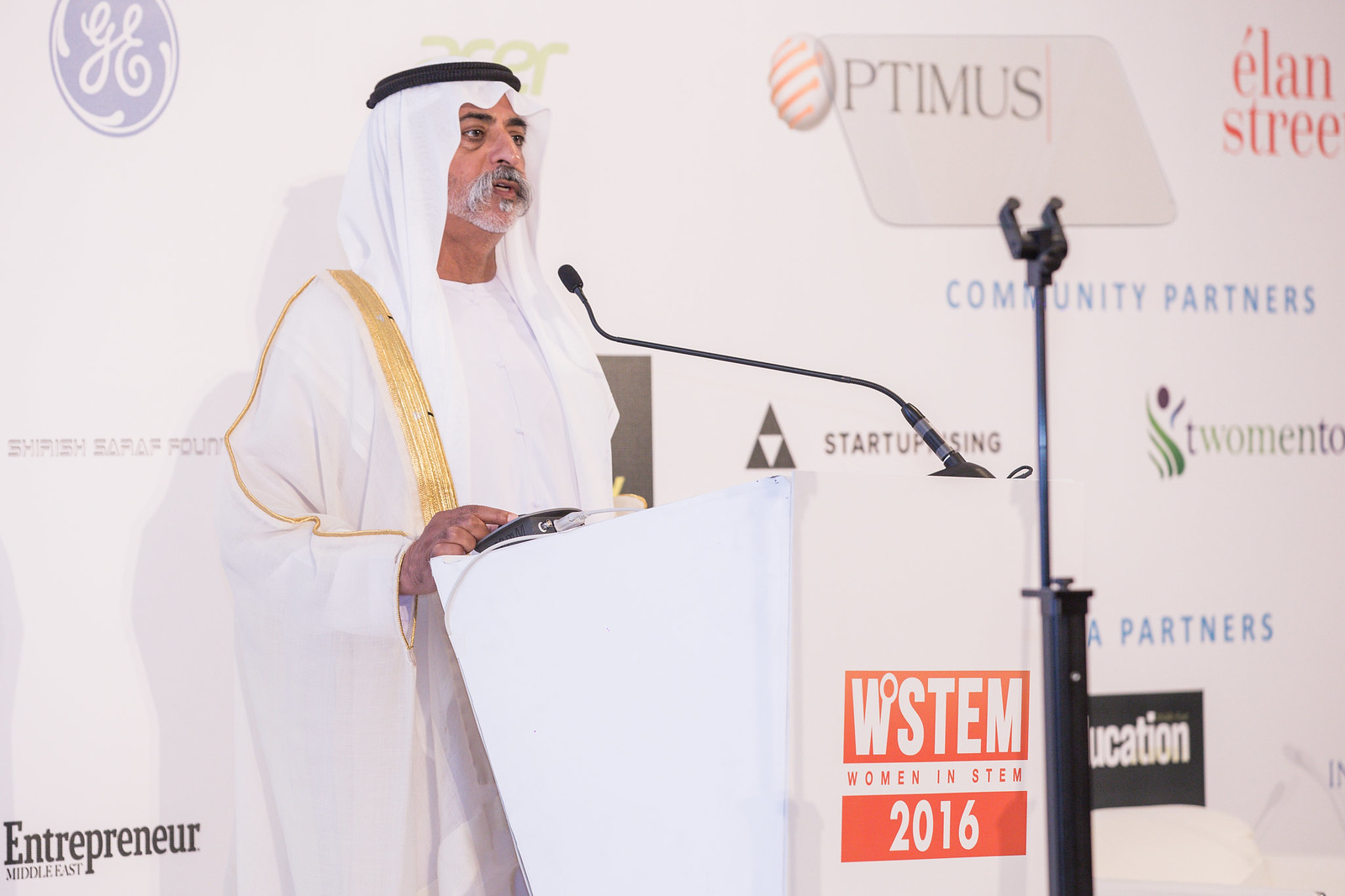The image depicts an older Middle Eastern man, perhaps in his 50s or 60s, standing behind a white podium adorned with two red bars. He is dressed in a white robe accented with gold trim and wears a white headscarf secured with a black band. His graying mustache adds to his distinguished appearance. A thin black wire microphone, with a fuzzy black end, extends up to his chin from the podium. The podium bears the text "WSTEM 2016" in white letters on a red background, with "Women in STEM" also prominently displayed. In his hand, he holds a small box connected to the microphone system. The background features a white wall covered with logos of various sponsors, including GE, Community Partners, and Optimus, indicating the venue to be a science or technology convention. The man is captured in a three-quarter angle, looking straight ahead, seemingly engaged in delivering a speech.